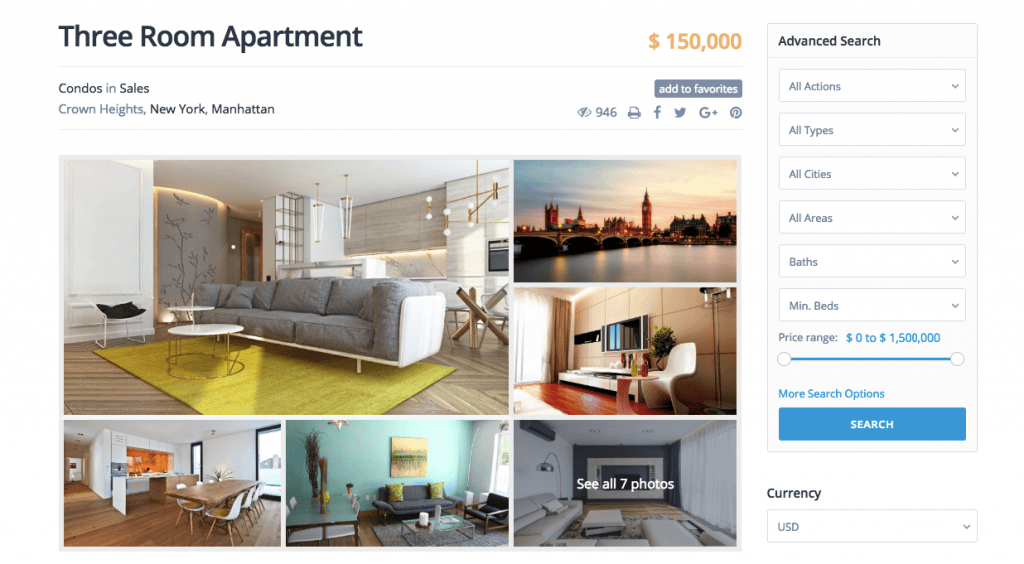A listing for a three-room apartment priced at $150,000 is showcased on a website with a clean, white background. The price is emphasized in orange. Located in the vibrant neighborhood of Crown Heights, New York, this property is part of the bustling Manhattan real estate market. The main image prominently features a contemporary-designed living room with a gray couch and a striking yellow carpet. Supplementary smaller images include an illuminated New York City skyline at sunset, interiors of modern apartment rooms, a stylish dining room, and a cozy sitting area. Completing the visual tour, the last image on the right invites users to view all seven available photos, displayed in gray with white text. The webpage also highlights an advanced search feature, offering customizable options such as property actions, types, cities, areas, and minimum bedroom requirements, allowing users to refine their search criteria.